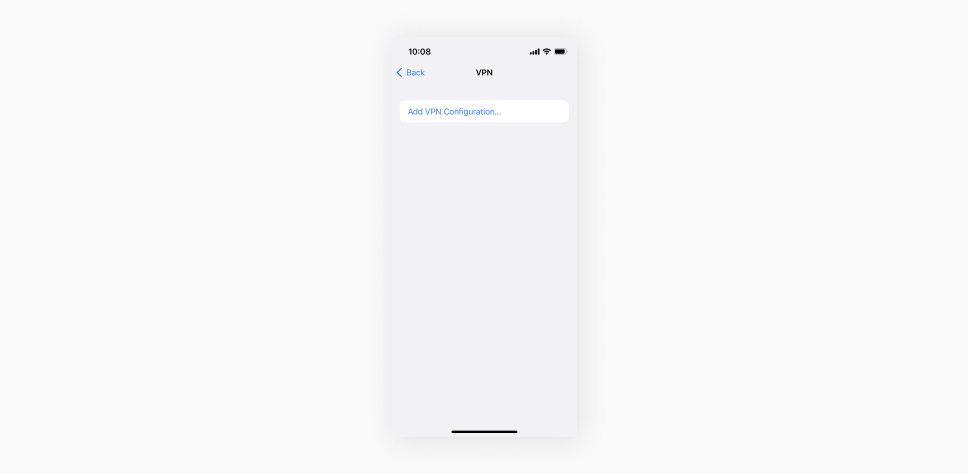In this simplistic image, which resembles the size of a phone screen, the background is a very light gray. At the top-left corner, the time is displayed in black numbers, showing 10:08. On the top-right corner, there are a series of icons indicating the phone’s status: the signal bars showing full connectivity, a signal strength indicator, and a nearly full battery icon. Below the time, a blue "Back" label with an arrow pointing left is positioned. In the middle of the screen, "VPN" is written in black letters. Below this, a white rectangular box features the text "Add VPN Configuration" in blue. The bottom of the image is marked by a centrally positioned black line, reminiscent of the speaker area on a phone, although the actual phone is not depicted.